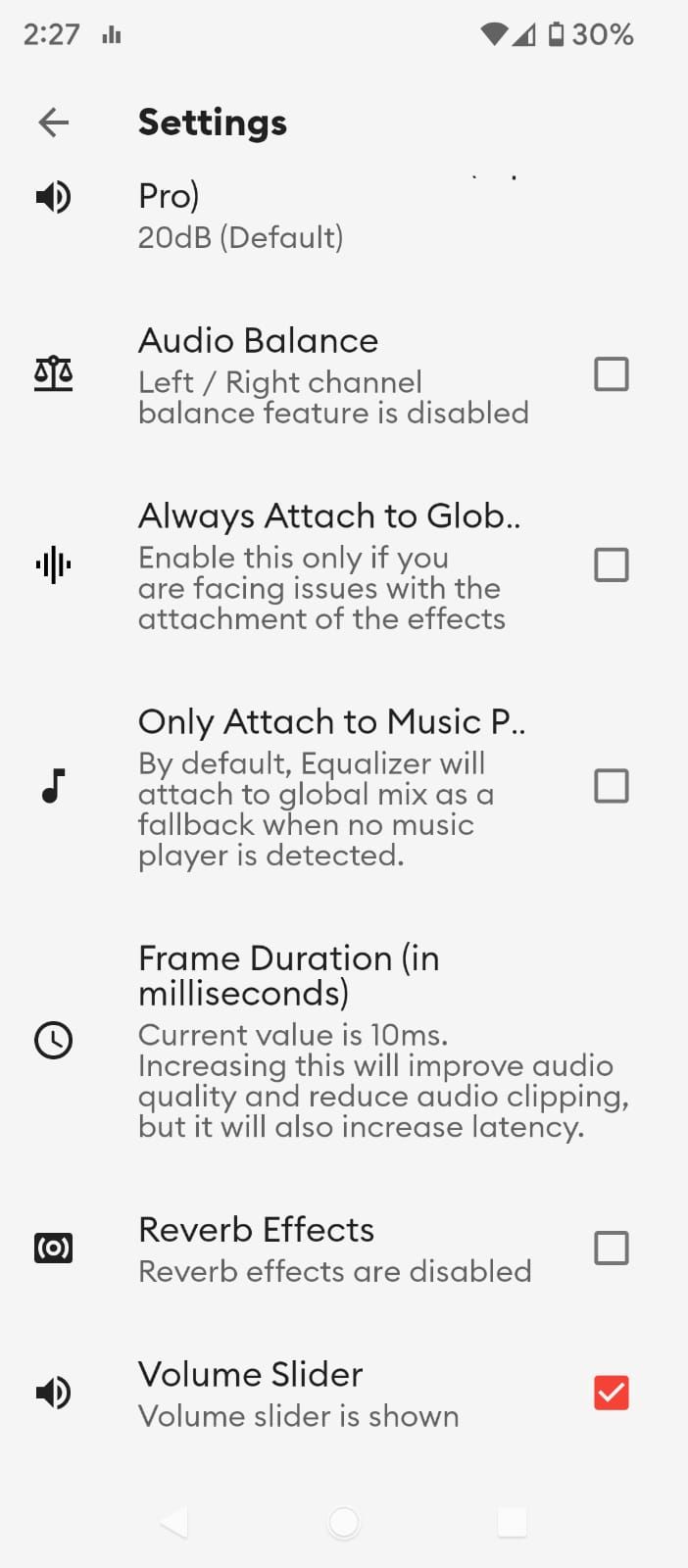This screenshot appears to be captured from either a tablet or a smartphone, showcasing a settings interface typically associated with an audio configuration application. The screen captures the device's status indicators and a detailed list of customizable audio settings.

In the top left corner, the time is displayed as "2:27," but without an AM or PM indicator, it might imply the use of military time. Adjacent to the time, a small graph is visible, providing additional contextual data. On the screen's right side, the status of various system utilities is shown: a fully active Wi-Fi symbol, a cellular signal at three-fourths strength, and a battery icon indicating it is at 30% capacity.

Beneath these indicators, a gray arrow points to the bold text "Settings." Following this, a bold speaker icon emits bent lines, accompanied by the text "Pro" on the right side. Below in gray text, it shows "20db" and "(default)."

Next, a bold black scale icon appears, followed by bold black text reading "Audio Balance." The subsequent gray text explains, "Left/Right channel balance feature is disabled." This section has multiple options, each accompanied by unselected squares except the last one. Underneath these settings, several bold lines of text state, "Always attached to global…" An explanatory note below mentions, "Enable this only if you are facing issues with the attachment of the effects."

Moving down, a music symbol accompanied by the text "Only attach music p…" is displayed. An additional note reads, "By default, the equalizer will attach to global mix as a fallback when no music player is detected."

A clock icon with adjacent text reading "Frame Duration (in milliseconds)" follows. Currently, the set value is "10 milliseconds," with a cautionary note that increasing this value will enhance audio quality and reduce audio clipping, albeit at the cost of increased latency.

Subsequent to this, there's a black square icon embossed with two bent lines and containing a white circle in its center, labeled "Reverb Effects." Under it, the status "Reverb effects are disabled" is displayed.

Finally, a speaker icon reappears with bent lines, labeled "Volume Slider," indicating that the volume slider is shown. The last option is checkmarked, turning the square orange with a white checkmark.

This descriptive caption provides a comprehensive overview of the interface presented in the screenshot, aiming to offer clarity and detail suitable for a detailed explanation.